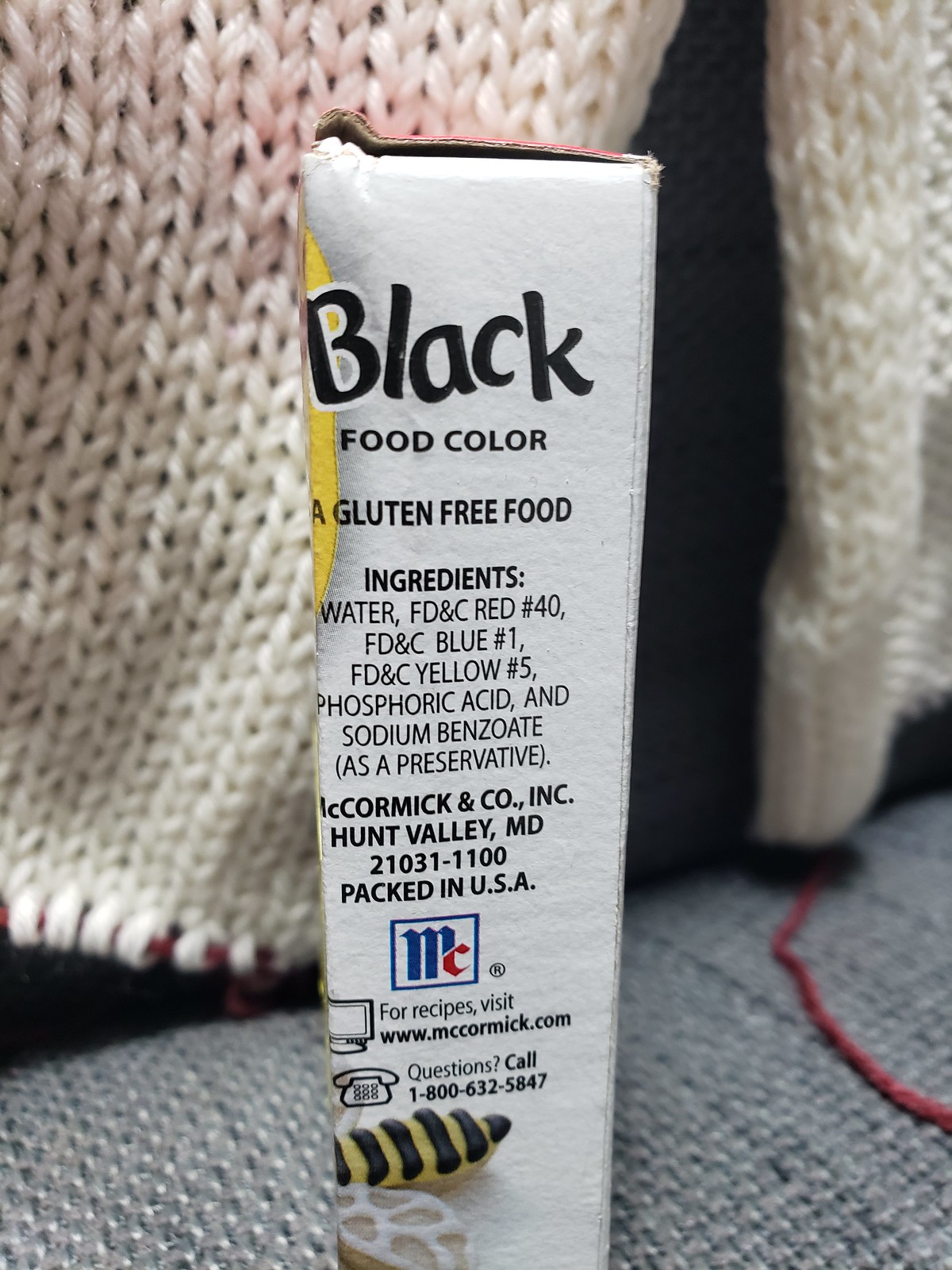In this photo, a cozy knitting scene is set against a fabric background featuring a knit texture. A white knitting project is in progress, with yarn strewn across what appears to be the cushion of a chair. The chair's fabric is gray on the bottom, contrasting with the cream-colored knitting happening in the background. Positioned in the lower left corner is a knitting needle, hinting at the ongoing creation. In the foreground, a package of McCormick black food coloring stands prominently. The packaging details that it is gluten-free and lists its ingredients: water, coloring agents (blue, yellow), phosphoric acid, sodium benzoate, and preservatives. The package highlights that it is distributed by McCormick Incorporated, based in Hunt Valley, Maryland, and packed in the USA. It also features the McCormick logo and includes an invitation to visit McCormick.com for recipes. For inquiries, a contact number 1-800-632-5847 is provided.